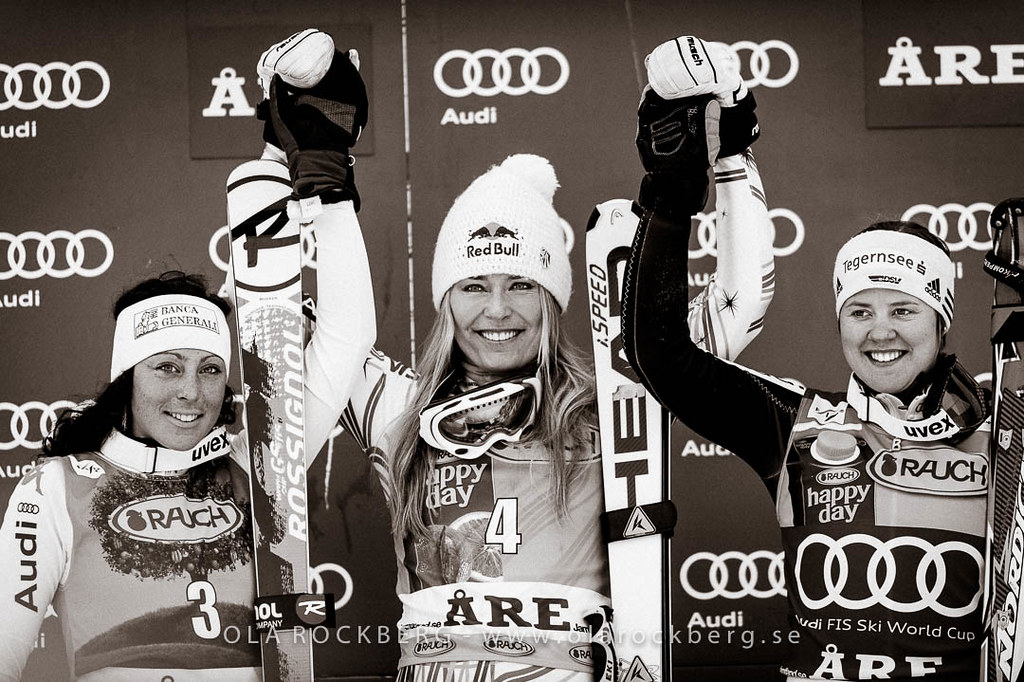In this black and white image, three female skiers stand side by side, posing for the camera. The central figure, who is the tallest, wears a white stocking cap emblazoned with "Red Bull" and has ski goggles around her neck. Her ski jersey features the number four, "Happy Day" in the upper left corner, and "A.R.E." on her stomach. She holds up the arms of the two skiers beside her. The skier on the far left sports a white bandana that reads "Thank a General" and a jersey with "R.A.U.C.H." and the number three on it. Her jersey also has "Audi" on the left side of her arm. The skier on the far right dons a white bandana that says "Tenergyci" with "Adidas" slightly below. Her jersey also displays "Happy Day" and "R.A.U.C.H.", with circles and the text "Audi F.I.S. Ski World Cup" followed by "A.R.F." on her stomach. They all have their skis upright beside them. The backdrop features a black wall with the Audi logo and the word "Audi" beneath it, suggesting a sponsorship display. The image focuses primarily on the skiers and their detailed gear, filled with various sponsor logos.